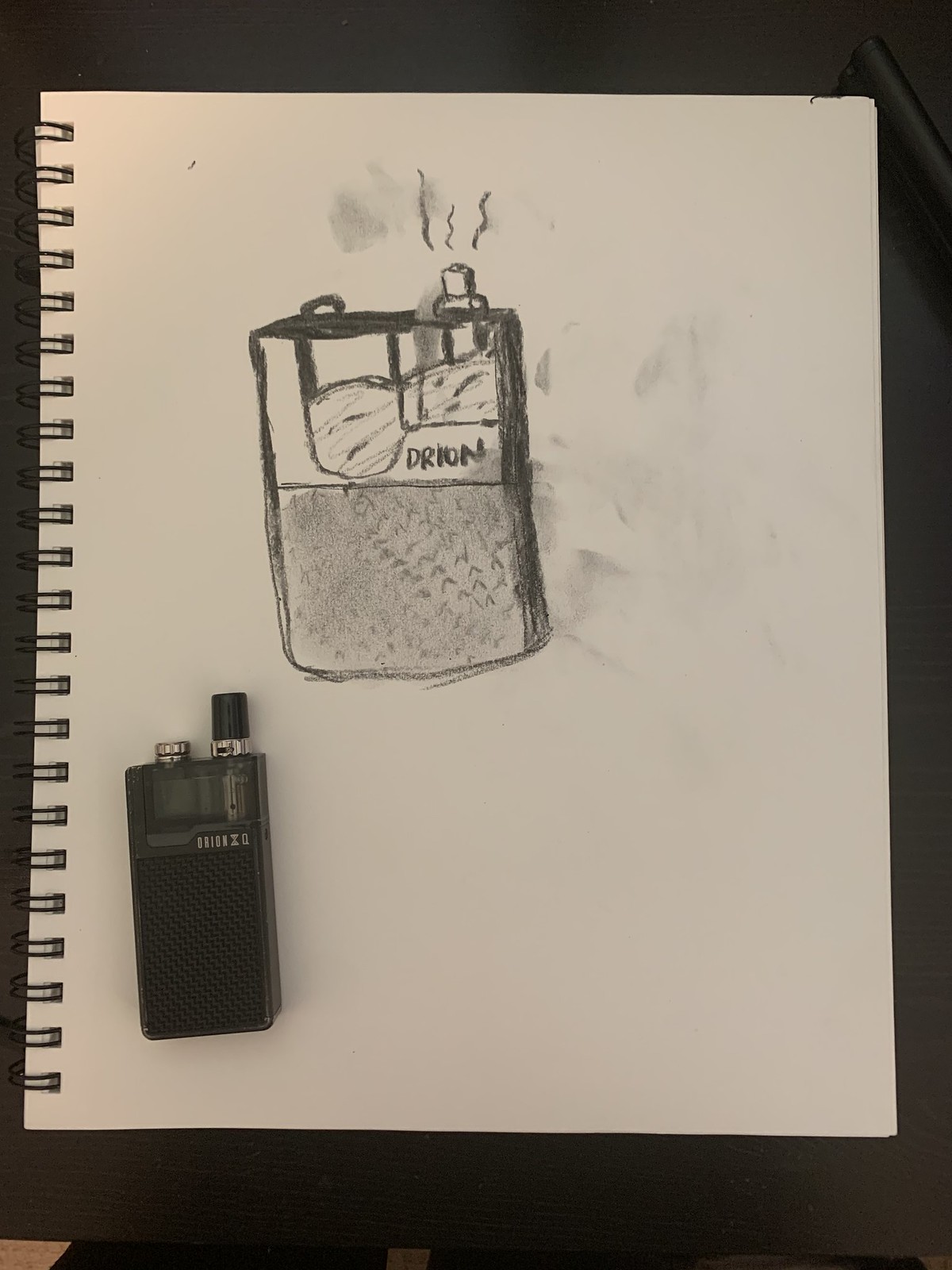The image captures a detailed drawing within a spiral-bound sketchbook, set against a black background. The sketchbook page features a meticulous pencil or charcoal drawing of a vaping device resembling a black, square, or rectangular perfume bottle. The device, modeled directly on the page, bears the brand name "Orion" (or "D-R-I-O-N"), indicating its identity. The sketch captures the device’s intricate details, including a lightly textured lower portion, transparent sections revealing the liquid inside, and dual spray or ignition points at the top. Above these features, fine lines simulate a spraying action. The device is mirrored in the sketch with realistic textures and precise labeling, blending seamlessly with the realistic portrayal of the actual object, which rests below the drawing as a reference model.